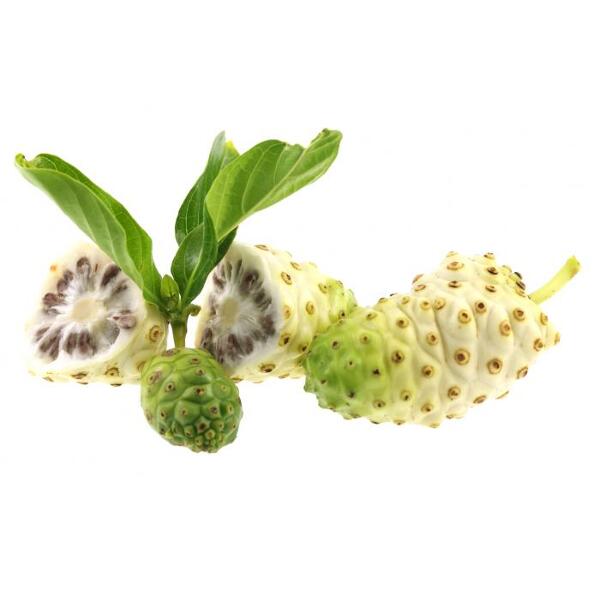This is a detailed colored image set against a white background, showcasing what appears to be an unusual fruit or vegetable in four different stages or forms. On the left, there's a green, immature version of the fruit with leaves sprouting vigorously from its top, almost resembling a green beehive. Beside it is a larger, similar fruit that has been sliced in half, revealing a white interior filled with black seeds organized in circular patterns. The exposed interior also has a darker, raisin-colored ring. On the far right, there is a larger version of the fruit, predominantly white with some green patches at the top, indicating it is not fully ripe. This version features yellowish, raised, bumpy pods or seeds on its surface, adding to its unique texture. The image collectively highlights the fruit's various stages of maturity and its intriguing internal structure.